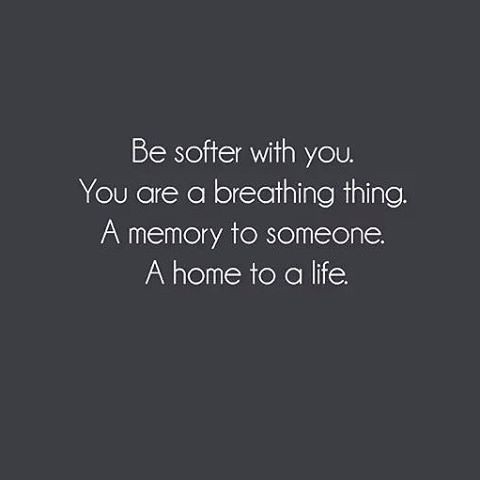The image is a square with a plain dark gray background that resembles wet cement, transitioning to black in some areas. Situated in the very center are four lines of white text, each line designed to be narrow and thin, and all text is centered. The font size appears to be around 15 or 16, striking a balance between not too small and not too large. The text reads: "Be softer with you. You are a breathing thing. A memory to someone. A home to a life." Each line is punctuated with a period, emphasizing their individual importance. There's more gray space at the bottom, creating a slightly uneven visual weight. The image exudes an inspirational vibe, resembling something that might be shared on social media platforms like Instagram. There are no people or additional elements present in the image, highlighting the simplicity and impact of the text alone.